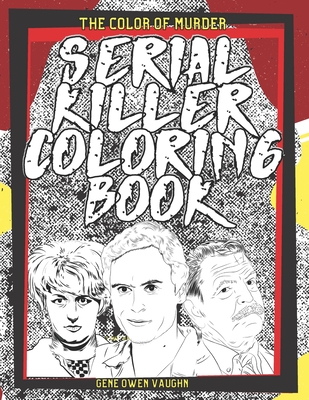The book cover, predominantly black and white, is titled "Serial Killer Coloring Book: The Color of Murder," authored by Jean Owen Vaughn. The central theme of the cover includes monochromatic illustrations and thick, white lettering that reads "Serial Killer Coloring Book" with a double-stroke style and marked holes within the text, giving it a worn look. 

The cover features three faces, each staring directly at the viewer, lined down the middle. On the left is a woman with short hair and a stern expression. In the middle is a younger man smirking slightly, while on the right is an older gentleman with a mustache, giving an inquisitive look. The background includes deep red and yellow patches, enhancing the eerie and ominous feel of the design. 

Encircling the cover is a black rectangular frame, and at the bottom of the page, written in yellow letters, is the author's name, "Jean Owen Vaughn." The design invites readers to fill in various murder scenes within the book, likely requiring an ample amount of red crayon.